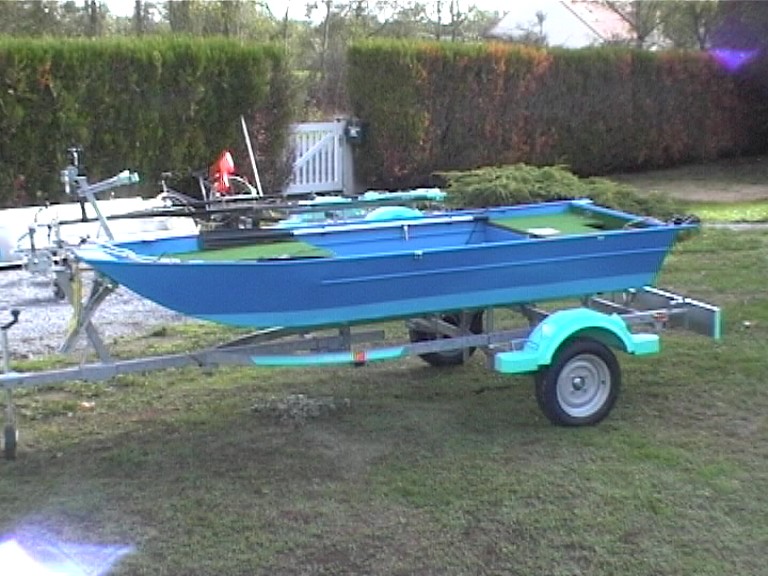This full-color daytime photograph captures a scene in the front yard of a house, distinguished by its well-maintained yet slightly color-changing tall green hedges and white picket fence gate with a diagonal bar. In the yard, patches of green and possibly snow-covered grass frame a small blue rowboat seated on a gray metal trailer featuring light blue wheel rims. The boat, which includes green seats and an indistinguishable small engine at its back, rests undisturbed. The absence of people adds to the peaceful static of the image, with a distant mailbox and some trees hinting contextually at a residential setting.